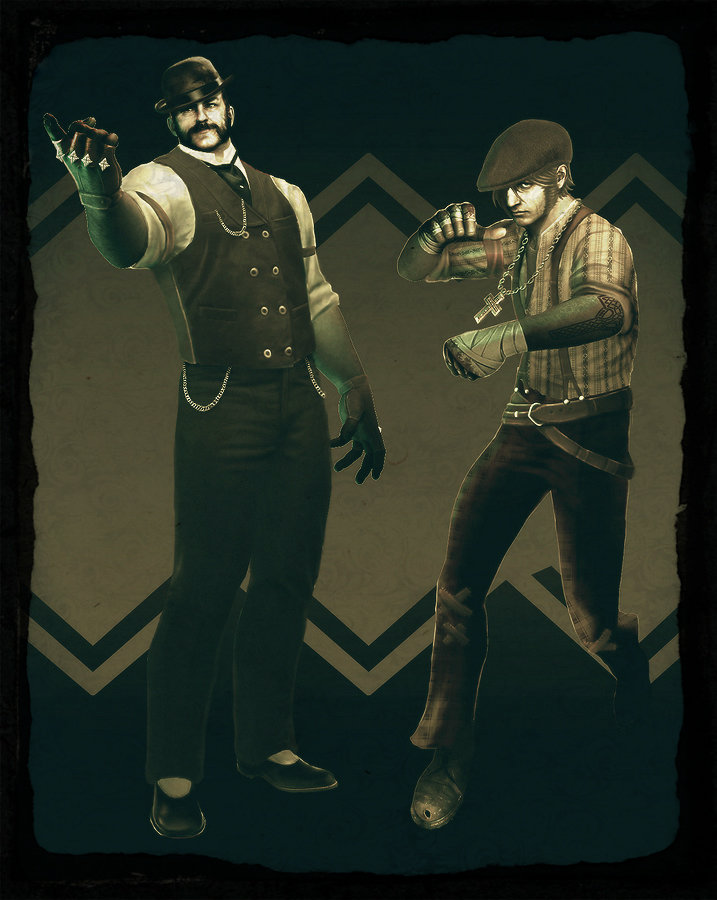This black and white illustration features two full-grown men dressed in early 20th-century attire, potentially professional boxers from the late 1800s to early 1900s. The man on the left, larger and distinguished, is adorned with a derby-style black top hat and sports mutton chop sideburns that merge into a mustache. His outfit includes a black vest with eight buttons, a white shirt with black armbands, and a gold chain leading to a pocket watch. His dark pants and black and white shoes complement his ensemble, and his right hand is extended upward, showcasing a black glove with silver diamond studs.

The man on the right, smaller in stature, is ready for a bout in a boxing posture with his fists wrapped in tape. He wears a beanie, a plaid shirt, a leather belt around dark pants, and black boots. His hair crosses his face, adding to his rugged appearance. The background is a mix of zigzag beige and dark forest green lines interspersed with a white geometric shape, enhancing the vintage and dynamic feel of the scene.